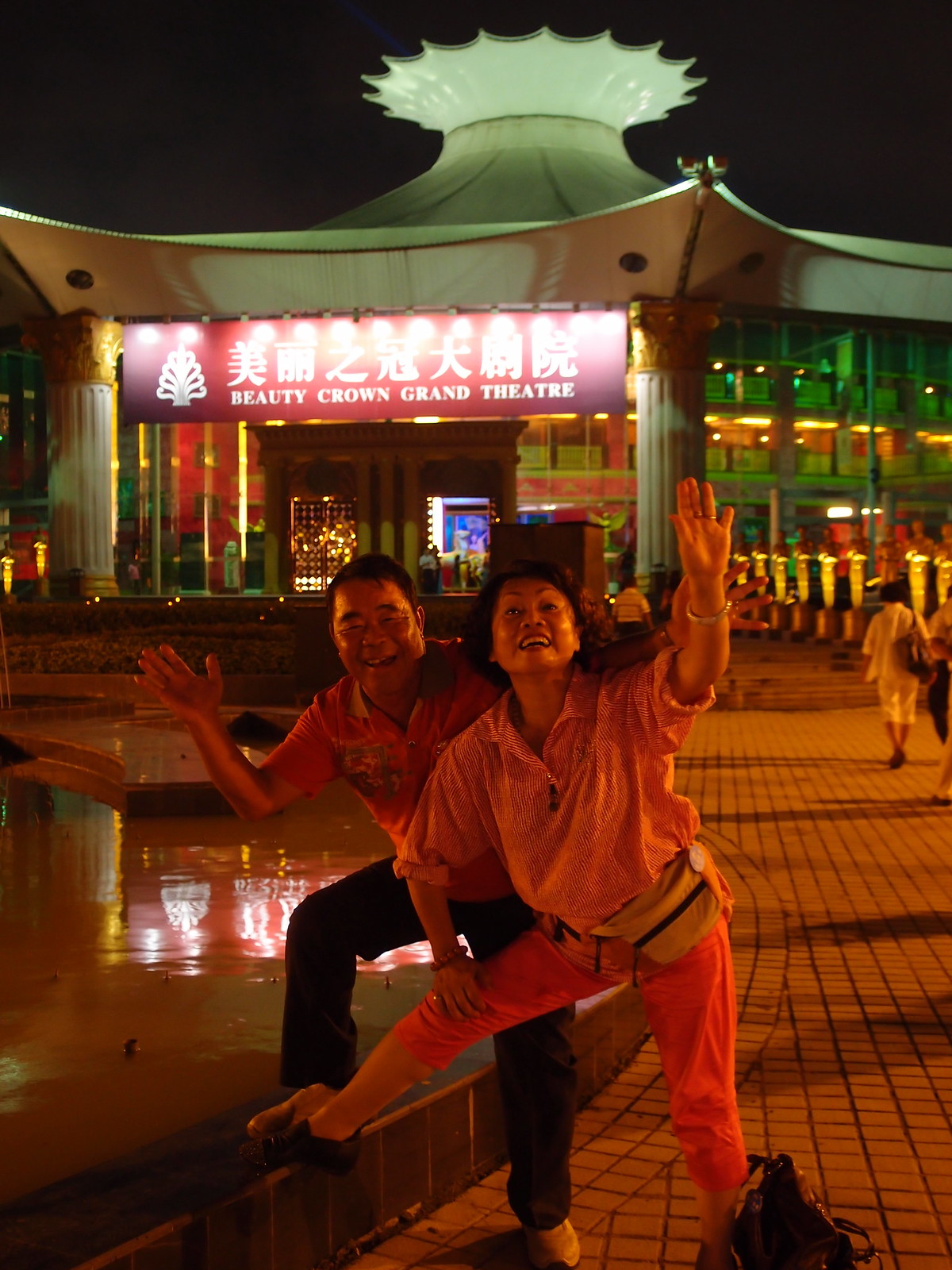This color photograph, though somewhat blurry and taken at night, captures an Asian couple joyfully waving at the camera in a bustling courtyard. The image is rectangular in horizontal alignment. They are positioned at the center, with a man on the left wearing black pants, a red collared shirt, and white shoes, and a woman on the right in pink pants, a pink shirt, black shoes, and a black and white fanny pack. Both appear to be in their fifties and of Asian descent, standing with one foot on the edge of a man-made pool, surrounded by a tiled walkway.

Behind them stands a striking white architectural structure with a distinctive pagoda-style design, topped by a circular sunburst ornament. This building, identified as the Beauty Crown Grand Theater, features a prominent sign with large Asian lettering in pink and purple, beneath which the title "Beauty Crown Grand Theater" is displayed in smaller white uppercase letters. Visible through the entrance are the illuminated and decorated interior and a concession stand.

The scene is vibrant with various colored lights, including green and yellow, reflecting off the building and the surrounding area, particularly highlighting a section with large windows, columns, and people walking on the pavered path to the right. The overall ambiance is festive and dynamic, capturing not only the joyful couple but also the lively atmosphere of the theater at night.